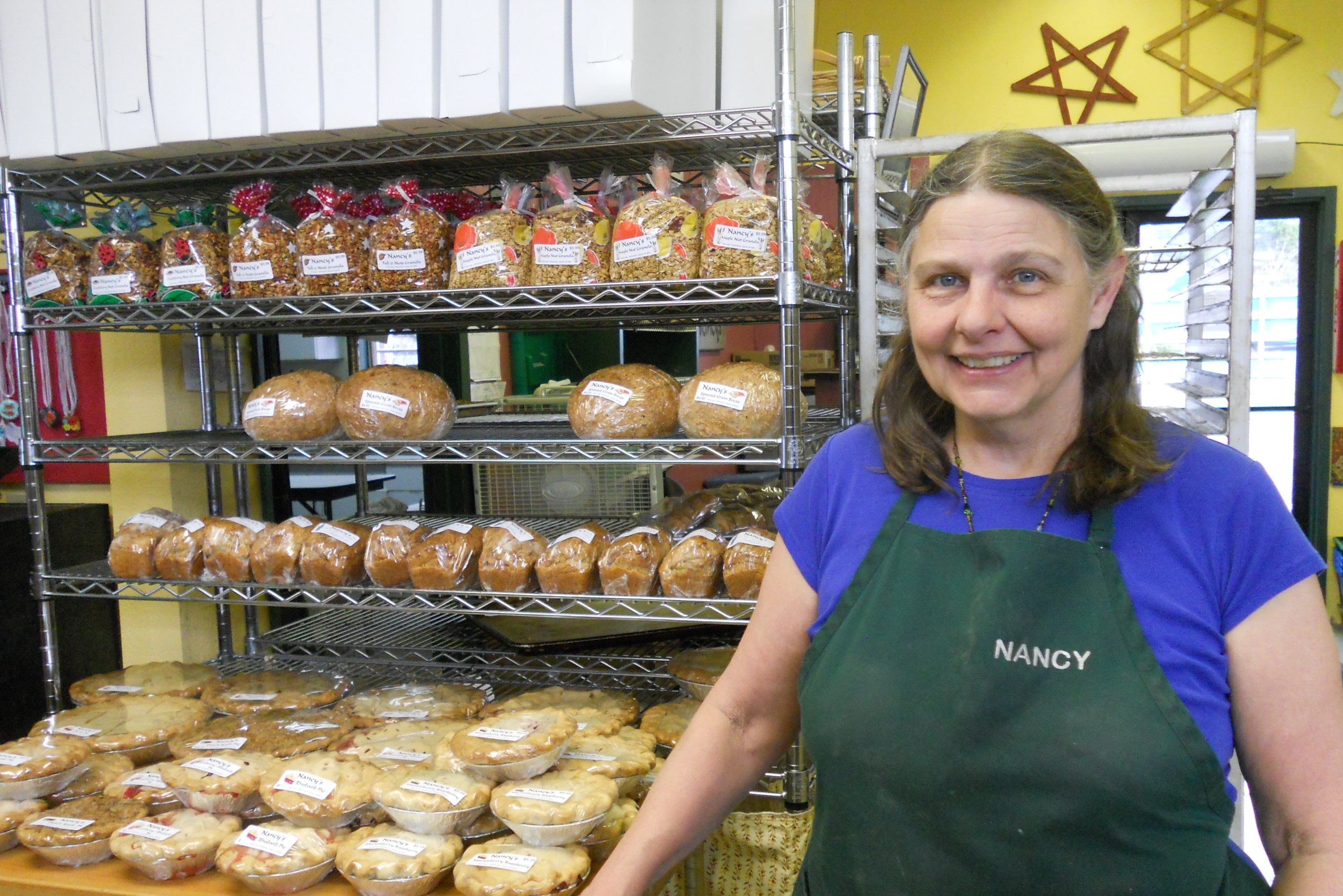In this detailed indoor daylight photograph, an older fair-skinned woman stands on the right, smiling warmly. Her shoulder-length hair is brown with subtle gray at the edges. She wears a short-sleeve blue shirt topped with a green apron that has the name "Nancy" printed in white letters. The woman is situated in what appears to be a bustling bakery.

She's positioned beside three metal racks filled with a variety of packaged baked goods. The bottom shelf holds an array of dark brown loaves of bread. The second shelf features four circular-shaped breads, possibly indicating their popularity given their scarcity. The top shelf displays square-shaped cakes, each adorned with a little bump or hilt at the top, and some are enclosed in black paper. Additionally, a table is in front of these racks, showcasing plastic bowls filled with circular light yellow pastries and some darker brown ones on the left.

Further details in the background include metal trays, a doorway leading outside, and a yellow wall adorned with stars. Another doorway on the left appears to lead to a different room within the establishment, completing this bustling bakery scene.